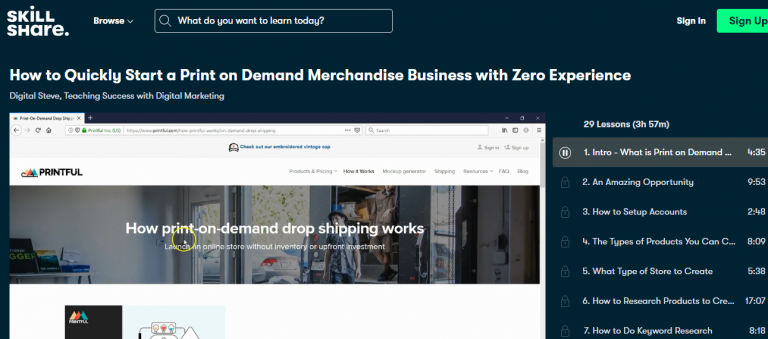A screenshot of the Skillshare website prominently displays various navigation and user interface elements. At the top left corner, there is a drop-down menu labeled "Browse," allowing users to explore different categories of courses. Adjacent to it, a search bar asks, "What do you want to learn today?" inviting users to type in their learning interests. Towards the right side of the header, options to "Sign In" or "Sign Up" are clearly visible.

Central to the image is a featured course titled "How to Quickly Start a Print-on-Demand Merchandise Business with Zero Experience," taught by Cole Steve, an expert in digital marketing. Within the website, another search input is partially visible, blurry, and indicates the term "Printful." Nearby, a menu lists various subcategories: "Products and Pricing," "How It Works," "Mock-Up Generator," "Shipping," "Resources," and "Blog," also featuring "Sign In" and "Sign Up" options.

The main image within the layout depicts a well-lit office setting with multiple windows. Outside the windows, a few cars are visible, suggesting the office overlooks a parking lot. Accompanying the visual, text explains, "How Print-on-Demand Drop Shipping Works: Launch an Online Store Without Inventory or Upfront Investment." On the right side of this section, a column details the course's structure: "29 Lessons," totaling "3 hours, 57 minutes." Various lesson selections are indicated below this summary.